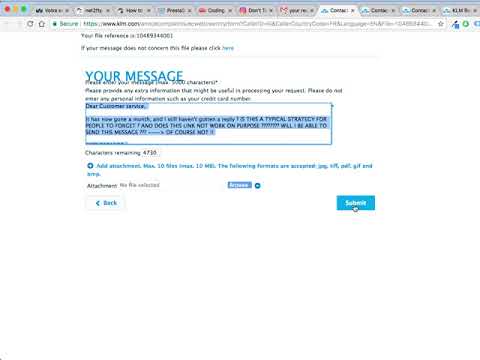This image is a detailed screenshot of a form submission page for a customer service or support request. At the top, there is a reference number used for tracking the submission. The form is titled "Your Message," and a note advises users to provide only relevant information to assist in processing their request while cautioning against including sensitive information, such as credit card numbers.

The main text area begins with "Dear Customer Services," followed by a detailed message. The user mentions someone named Gary who is experiencing hunger and is inquiring about typical strategies to address this issue. They also seek advice on what steps to take if the problem persists after the first attempt.

Below the message box, a character count indicates that 478 characters remain, suggesting a text limit. There is also an option to add attachments, with a maximum file size of 10 megabytes, supporting formats such as GIF, JPEG, and PDF.